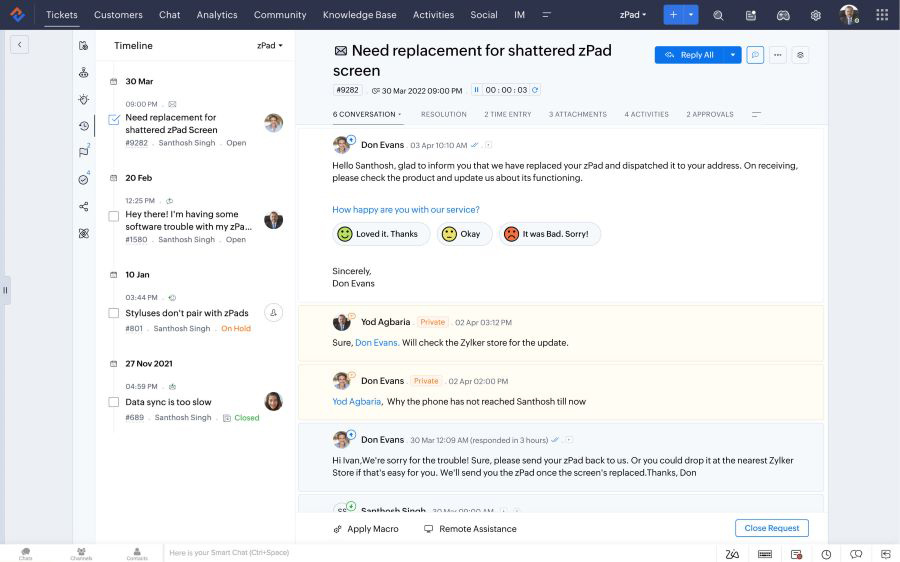**Detailed Caption:**

The screenshot displays a user interface with a horizontal black menu bar spanning across the top of the image. On the left corner of the menu bar is an icon. The text on the menu bar is light gray and includes the following options: "Tickets" (which is underlined), "Customers," "Chat," "Analytics," "Community," "Knowledge Base," "Activities," "Social," and "IM." On the right side of the menu bar, the word "Pad" is displayed. Adjacent to it are two blue squares; the one on the left has a white plus sign, and the one on the right has a white minus sign. Additionally, there are various icons aligned along the right edge of the bar.

Below the menu bar, the background is light gray. In the upper left-hand corner, there is an outlined gray box featuring a left-pointing arrow resembling a sideways "V." To the right of this box, a white rectangular panel extends down the page. Attached to the left side of this panel is a thinner, vertically-oriented strip in light blue, containing a series of icons.

In the main white panel to the right, there is a list formatted as a timeline. Starting with "30 MAR," each entry includes a checkbox. For example, an entry reads: "Need replacement for shattered iPad screen," which is checked off. Further down, there's another entry dated "20 FEB" that says, "Hey there, I'm having some software trouble with my," which remains unchecked.

To the right of the timeline list, there is a large blue square. At the top left of this section is a letter icon. Adjacent to it, in bold black text, is the statement, "Need replacement for shattered Z-pad screen." On the right side of this statement is a blue "Reply All" button with a dropdown menu, accompanied by additional icons like an ellipsis and a settings gear.

Below this section, comments from various users are displayed in a specific format: each comment includes a profile image on the left, the person's name to the right of the image, and the comment text below the name.